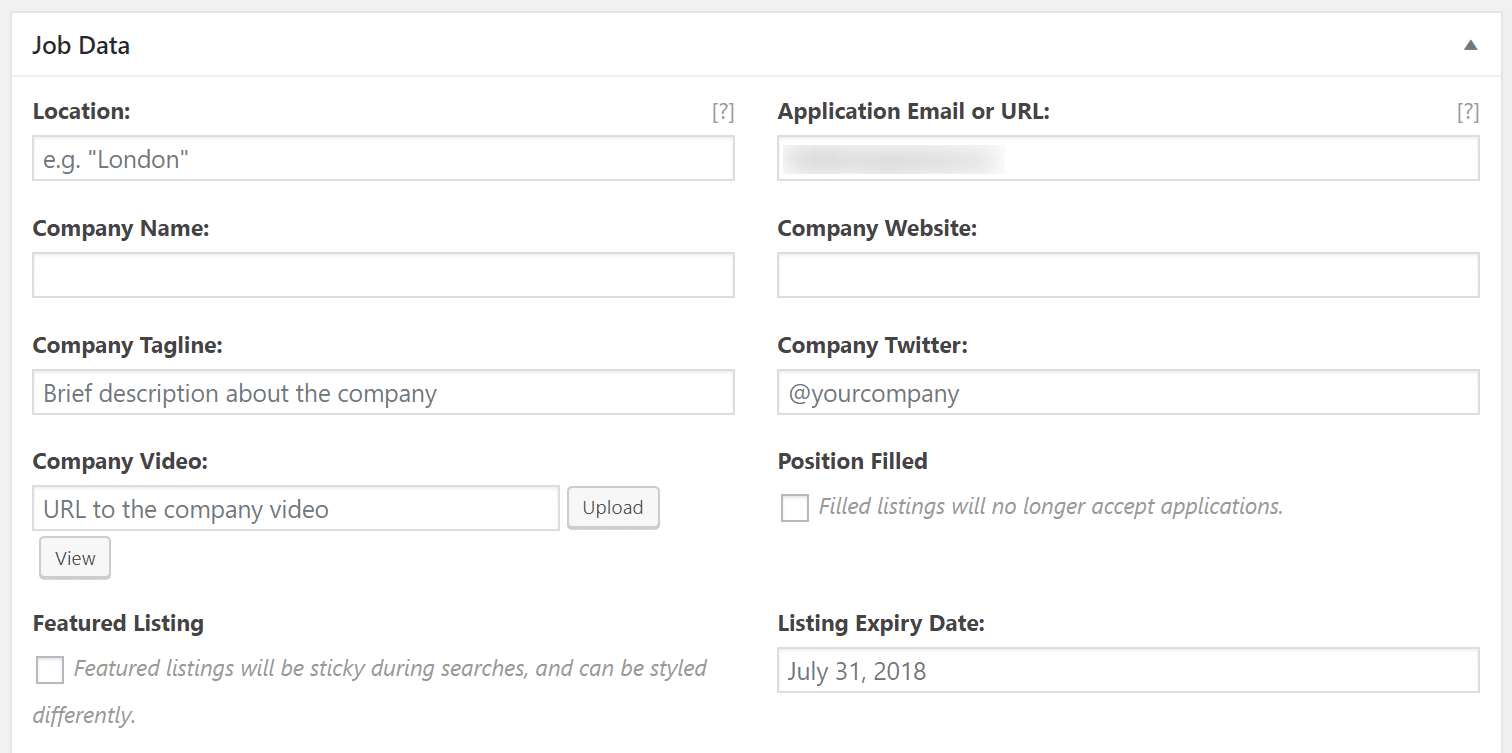In this image, we see a structured job data form with a gray border and a white interior. The form consists of several fields designed to be filled out with relevant job information. At the top, in bold black text, it reads "Job Data." Below this, there are various labeled sections:

1. **Location:** This section provides an example text, such as "London," to guide the user.
2. **Company Name**
3. **Company Tagline:** Includes example text stating "brief description about the company."
4. **Company Video:** Contains a placeholder "URL to the company video" and features both an "Upload" and a "View" button.
5. **Featured Listing:** An option to check, with an explanation that a featured listing will be sticky during searches and can be styled differently.

On the right side of the form, additional fields are displayed:
   
6. **Application Email or URL:** This field is grayed out.
7. **Company Website**
8. **Company Twitter:** Displays an example handle, "@yourcompany."
9. **Position Field:** Includes an option to check, indicating the listing will no longer accept applications.
10. **Listing Expiry Date:** The box shows a date, "July 31st, 2018," which could be real or just an example.

Overall, the image depicts a simple yet comprehensive form meant for entering job-related data and various company details.